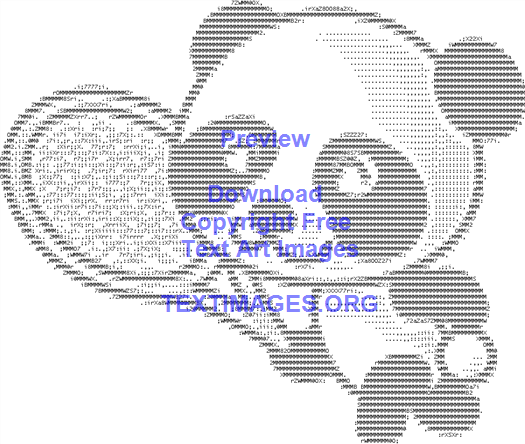The image depicts a creatively designed, animated panda bear holding a tennis racket, walking towards the left. This pixelated artwork uses a grayscale palette, with darker shading around the eyes and ears, transitioning to lighter shades on the left side of the head to provide depth and a realistic effect. Crafted using a combination of keyboard characters such as numbers, letters, and symbols, the bear appears to be carrying a tennis ball in its left paw while holding the racket in its right. Overlaying the bear is blue-purple text that reads: "preview, download, copyright-free text art images, textimages.org," with the last part written in all caps. This image is a unique blend of text art and digital creativity.